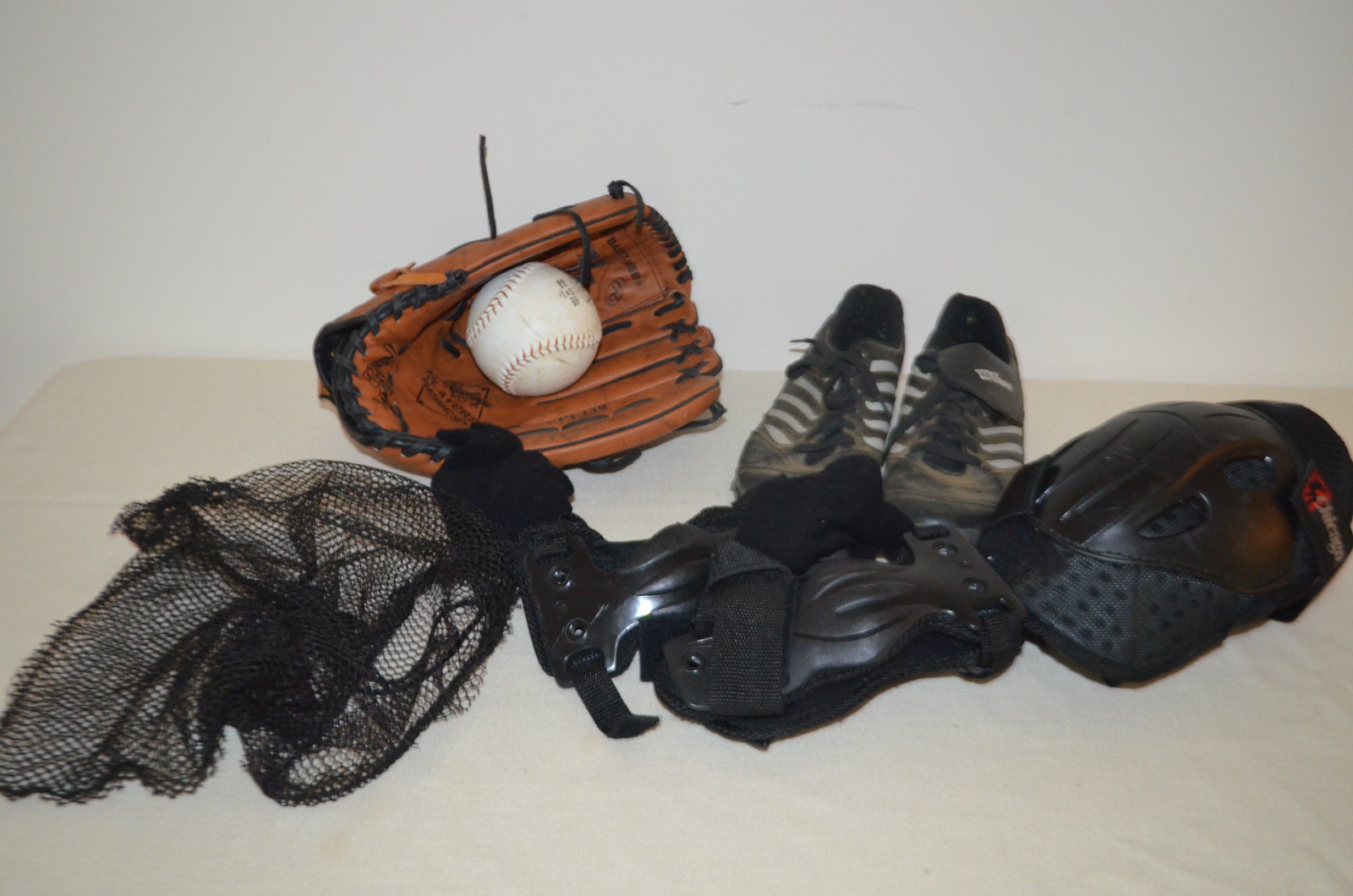This photograph captures a meticulously arranged collection of baseball equipment, set against a light gray, slightly smudged wall. Laid out on an off-white, slightly rumpled rectangular table, the ensemble prominently features a brown baseball glove on its side, cradling a white baseball at the lower portion of the frame. To the left of the glove, there is a piled black net, likely a jersey, indicating team identification. Below the glove lies protective gear, possibly comprising a chest plate and knee or neck pads, constructed from hard black plastic—suggesting use by a catcher. Above this protective equipment is a pair of well-worn black cleats with white stripes, positioned with their soles facing the chest plate. Further to the right of the cleats, there is a black hard hat helmet, completing the assembly of gear essential for a baseball player.